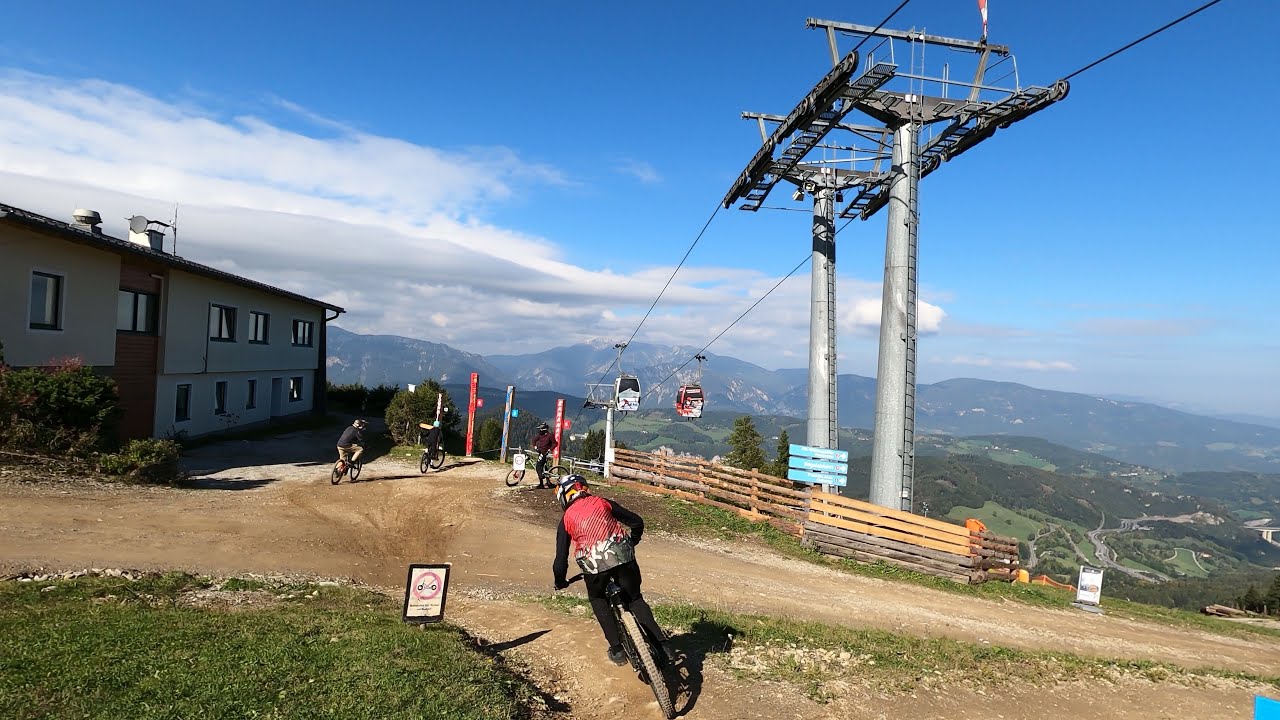This image captures a vibrant mountain biking scene in the summer, set against a picturesque mountainous backdrop. At the center-bottom of the image, a mountain biker clad in a long-sleeved black shirt, with a red mesh tank top and a multicolored helmet, prepares to embark on a dirt path that stretches horizontally across the frame. This path, made of brown dirt, splits lush green grass on either side. Three other bikers are positioned at the top of the path, further into the image, one of whom is next to a 'No Golf Carts' sign.

To the left of these riders stands a house–or possibly a clubhouse–constructed with red bricks and tan accents. To the right, two brightly colored gondolas, painted in greens and reds, move along gray cables supported by tall, silver poles, part of the lift structure that transports them up the mountain. People and bikes appear diminutive in comparison to the vast landscape surrounding them.

In the background, rolling hills and majestic mountains, some still sprinkled with patches of white snow, rise against a clear blue sky. The scene is bathed in sunlight, indicating a bright, sun-drenched day, despite the fluffy clouds hovering above. Pines and other trees pepper the distant hills, completing this stunning, action-filled portrayal of a day of mountain biking adventure.